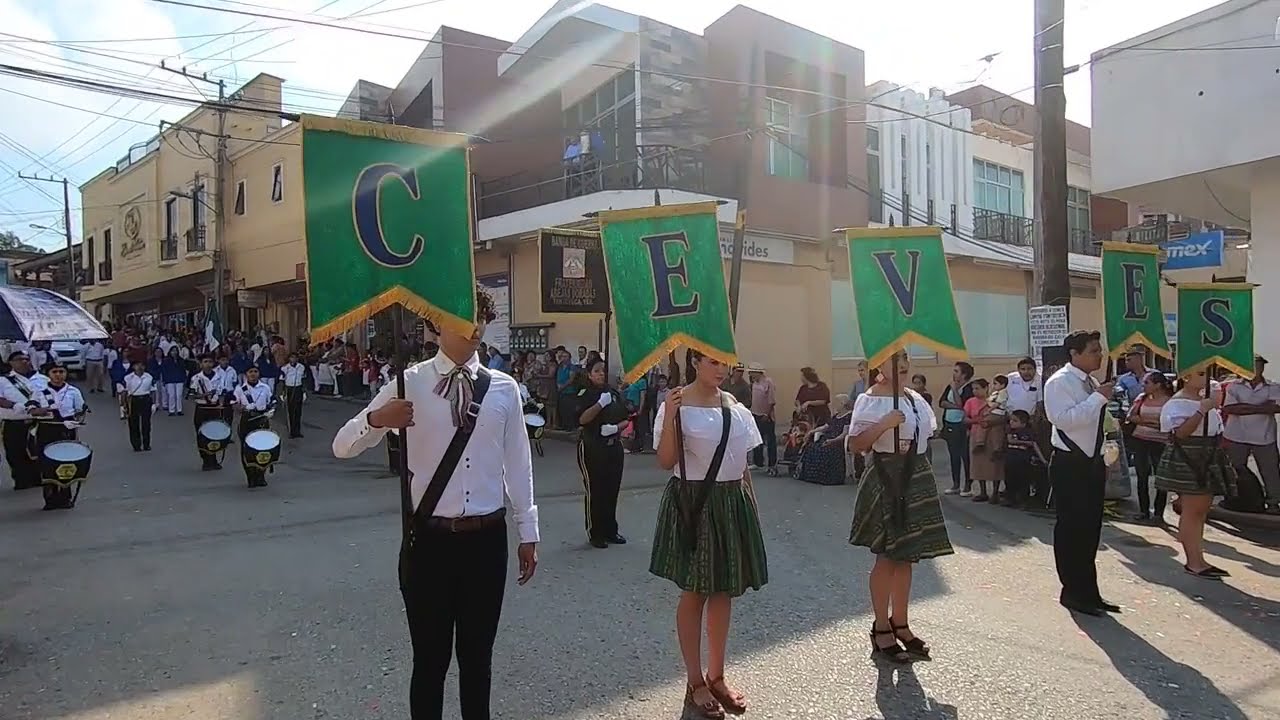This horizontally aligned rectangular image captures a lively downtown parade scene. In the forefront, five individuals are positioned in a row at the center of the image, each holding a green and gold-trimmed banner with a blue letter, spelling out "C-E-V-E-S" from left to right. The men, dressed in long-sleeved white button-down shirts and black slacks, hold the 'C' and first 'E', while the women, adorned in white off-the-shoulder tops with sashes and green skirts, hold the 'E', 'V', and 'S'. The road beneath them is gray pavement, and flanking the parade route are spectators lined up on the sidewalks. The backdrop features two-story yellow and brown brick buildings, complete with numerous windows and black railings on the upper levels. Just behind the letter holders, a group of drummers dressed similarly in white shirts and black slacks march, their snare drums strapped to their waists. In the upper left corner of the image, a partly sunny sky with large white clouds is visible.